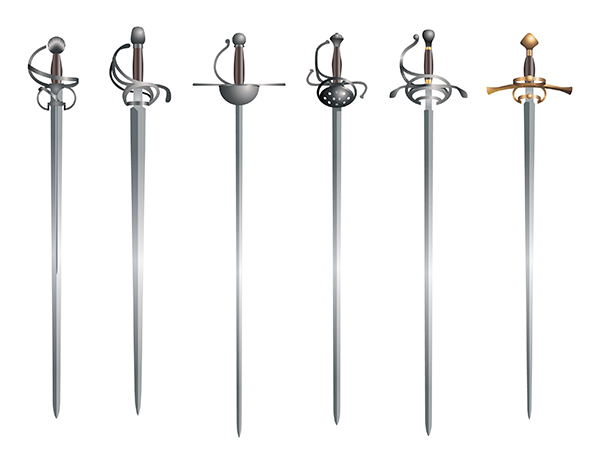The image showcases six upright swords against a white background, each boasting uniquely designed handles. The swords appear to be used for fencing or sword fighting, with differences primarily in their handles and blade widths. Three of these swords feature hand guards made of intricately swirling metal, presumably to deflect opposing blades and protect the wielder's hand. Another sword has a distinctive large cup at the hilt, while one has a cup with perforations resembling a colander. The last sword stands out with gold-colored embellishments, including a crossbar hilt design. Most of the swords are rendered in a muted silver hue, giving them a slightly pixelated, low-resolution appearance, except for the gold-accented sword which adds a touch of color contrast to the collection. The swords are approximately the same length, with slight variations making three of them a bit shorter than the others. The detailed and diverse designs of the hilts range from swirling and filigree to geometric motifs.